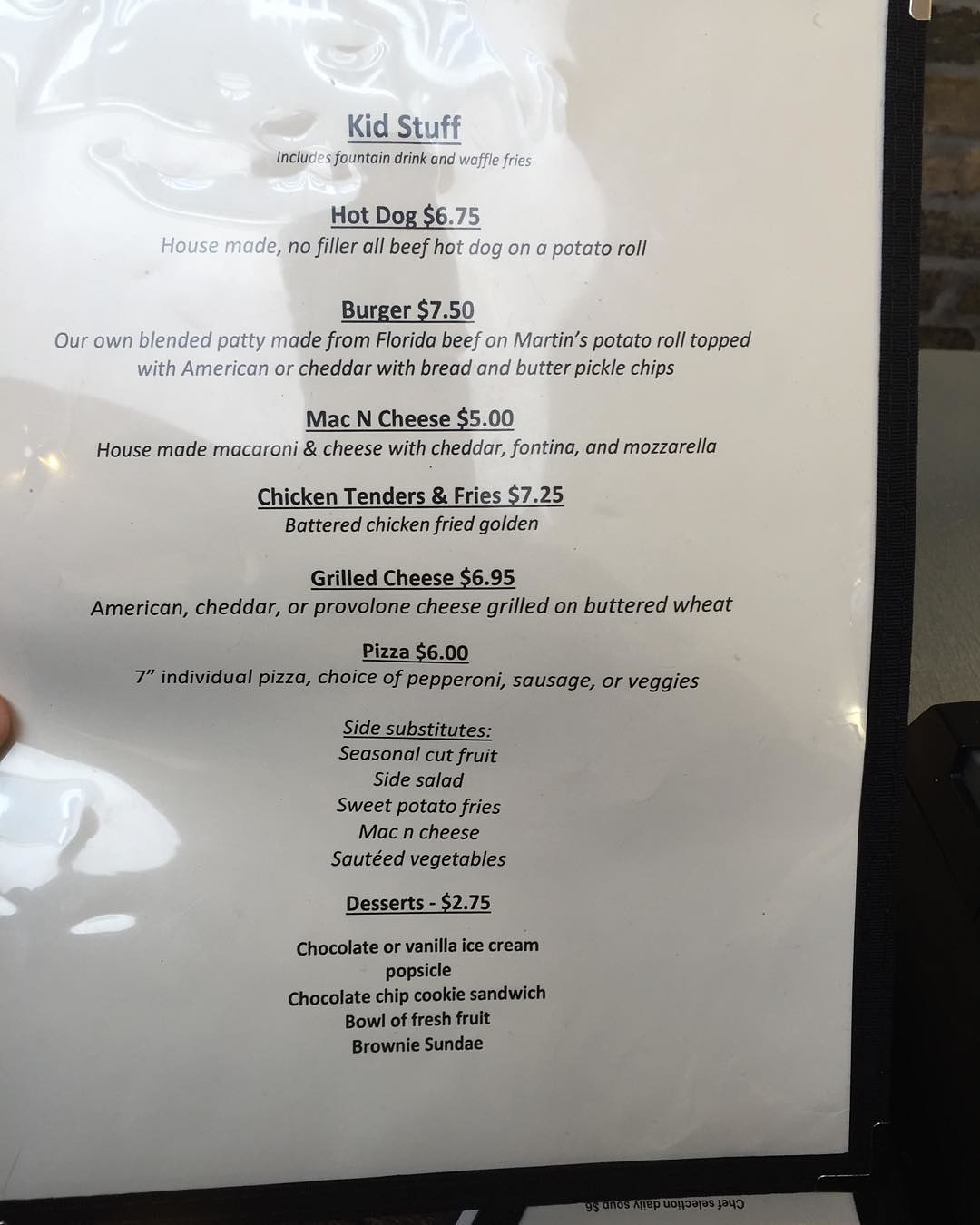This photograph showcases a children's menu elegantly displayed on a piece of white paper, neatly enclosed in a black menu holder. At the top, the section labeled "Kids Stuff" prominently stands out. Each entrée in this section comes with a fountain drink and waffle fries, ensuring a delightful meal for young diners.

The menu items and their prices are:

- **Hot Dog**: $6.75
- **Burger**: $7.50
- **Mac and Cheese**: $5.00
- **Chicken Tenders and Fries**: $7.25
- **Grilled Cheese**: $6.95
- **Pizza**: $6.00

For the pizza, children have options of pepperoni, sausage, or veggie toppings. The grilled cheese offers a choice between American, cheddar, or provolone cheese, all elegantly grilled on wheat bread. The mac and cheese boasts a rich blend of cheddar, fontina, and mozzarella.

Additionally, if waffle fries aren't preferred, there's a variety of side options available, including fruit, side salad, sweet potato fries, mac and cheese, or sautéed vegetables.

The dessert selection, priced at $2.75 each, includes:

- Chocolate or vanilla ice cream
- Popsicle
- Chocolate chip cookie sandwich
- Bowl of fresh fruit
- Brownie sundae

Each dessert promises a sweet ending to the meal. The menu's text is centered on the page, with each item highlighted in bold print, and brief descriptions provided underneath, ensuring a clear and appealing presentation for all choices.